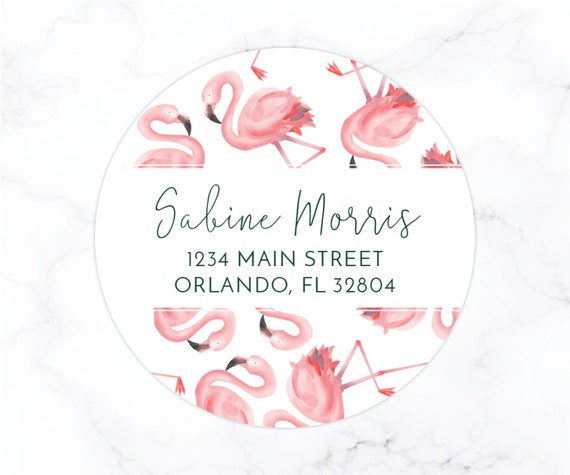The image is a circular sticker or possible coaster mock-up, featuring the name "Sabine Morris" in a cursive black font against a marble-patterned background. The text is set on a white strip running across the middle of the circle. Below the name, the address "1234 Main Street, Orlando, Florida 32804" is printed. The design is adorned with pink flamingos at the top and bottom of the circle, each bird characterized by a long S-shaped neck, a dark beak, and a mix of red and black feathers toward the end of its wings and tail. The flamingos appear to be the same image, mirrored and rotated to fill the space effectively. The overall aesthetic suggests it could be used for address labels, business card coasters, or other decorative purposes.